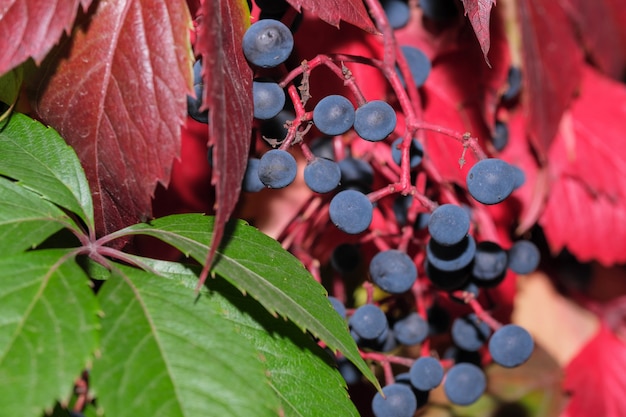This close-up photograph showcases a vibrant mix of leaves and berries. In the bottom left corner, large green leaves contrast sharply with the predominantly red foliage that fills most of the image. Among the leaves, which are elongated and vary from lush green to deep red, there are also distinct berries hanging from pinkish-red branches. These berries are round, blue to black in color, with a slightly flattened shape and a velvety texture. Despite being blurred, the background reveals an abundance of red leaves, adding depth and a rich tapestry of colors to the scene.